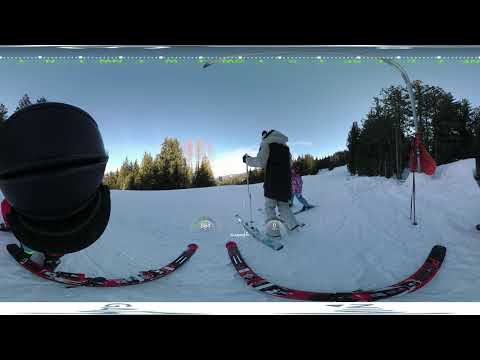The photograph captures a dynamic winter scene featuring an adult and a child skiing on a snowy hill. The adult skier, faced away from the camera, is clad in a black and gray jacket extending down to their thighs, paired with light gray ski pants. They hold at least one ski pole in their left hand and navigate the snow on white skis. To the right, a young girl, identified by her pink jacket and light blue pants, is slightly turned toward the camera while also on skis, indicating a family or teaching moment. At the bottom of the image, due to possible GoPro or body camera distortion, two curved skis, black and red, lie in the snow, adding to the immersive feel of the setting. The background is detailed with tall, green pine trees, alongside distant leafless trees visible through an overcast sky where clouds peek out. The snowy hill slopes gently downwards, framed by black letterbox borders at the top and bottom of the image.